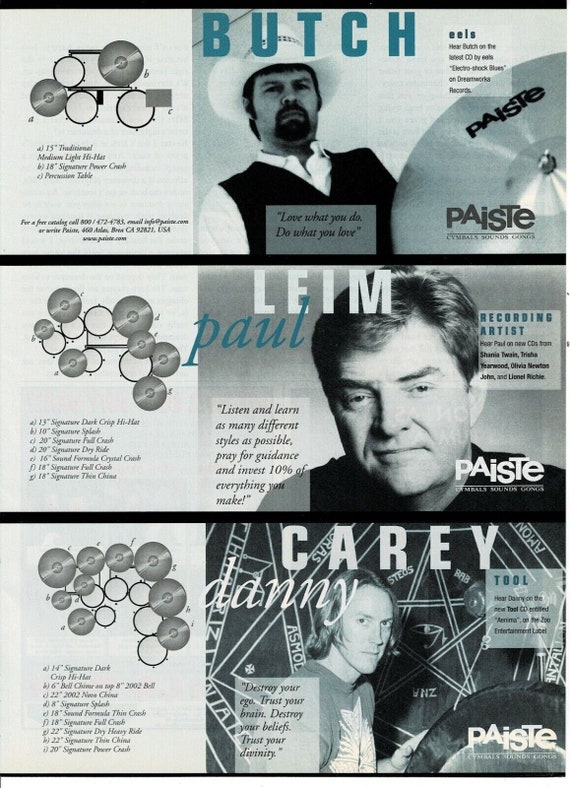The black and white magazine ad showcases three renowned drummers, each accompanied by their drum setup diagrams. At the top, a photo of Butch, who is dressed in a cowboy hat, white shirt, and black vest, stands next to a diagram of his drum kit labeled "ABC." His image is followed by a quote, "Love what you do, do what you love." The middle section features a photo of another drummer, Liam Paul, with his drum setup diagram nearby. His quote reads, "Listen and learn as many different styles as possible, pray for guidance, and invest 10% of everything you make." At the bottom, a photo of Danny Carey from the band Tool shows him at his drum kit, coupled with his distinctive quote, "Destroy your ego, trust your brain; destroy your beliefs, trust your divinity." Each section of the ad prominently displays the Paiste logo, indicating the use of their cymbals, sounds, and gongs. The ad is a tribute to the art and dedication of these drummers, expertly captured in a clear and naturally lit setting.